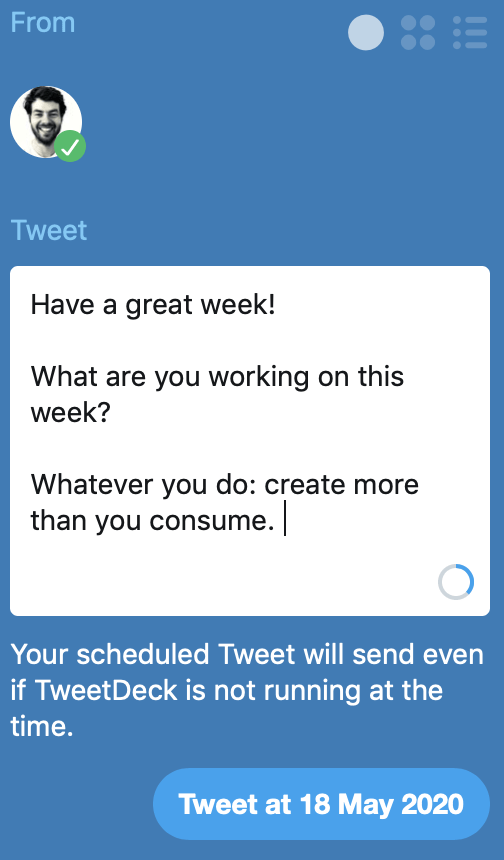A detailed caption for the described image could be:

"A screenshot of a scheduled tweet on TweetDeck, posted on May 18, 2020. The tweet message reads, 'Have a great week! What are you working on this week? Whatever you do, create more than you consume,' displayed in white text against a dark blue background. The image features a small circular profile picture on the bottom right, depicting a person with black hair resembling a 'discount' Seth Rogen, but not clearly showing their face. Below the tweet text, there's an indicator showing less than half of the character limit has been used. The top of the screen displays a menu bar with several options, including a pull-down menu, typical of the TweetDeck interface, which allows tweets to be scheduled for automatic posting even when the program isn't running."